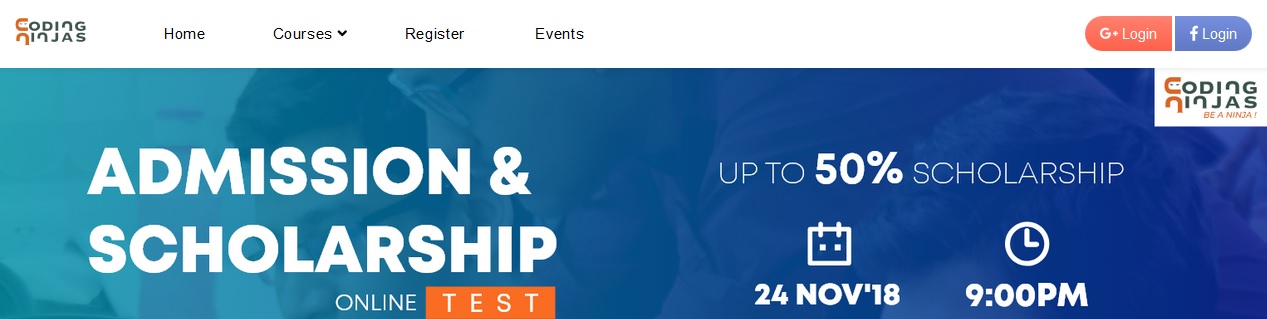The image appears to be a screenshot of a website layout, possibly an educational institution's homepage or landing page for prospective students. 

On the left-hand side, there is some text with the first letter in orange and the rest in black, though the exact text is unclear. Beneath this, there are navigation options labeled "Home," "Courses" (with a downward-pointing arrow indicating a dropdown menu), "Register," and "Events."

To the right, there's an orange shape containing a symbol and the text "Log In." Adjacent to this, there is a blue shape with the letter "F" and the words "Log In," possibly indicating a Facebook login option.

Below this, a larger blue box is visible. This box features a gradient from lighter blue on the left to darker blue on the right and seems to contain an indiscernible image. On the left side of this box, white text reads "Admissions and Scholarships," with the word "Online" situated underneath. 

An orange rectangle beneath this text has the word "Test" inscribed in it. To the right, the text "Up to 50% Scholarship" is prominently displayed, with an image of a calendar below it showing the date "24 NOV 18," and an icon of a clock with the time "9 PM."

In the upper right-hand corner of the image, there's a logo identical to the one on the top left-hand side, featuring letters where the first is in orange and the rest in black.